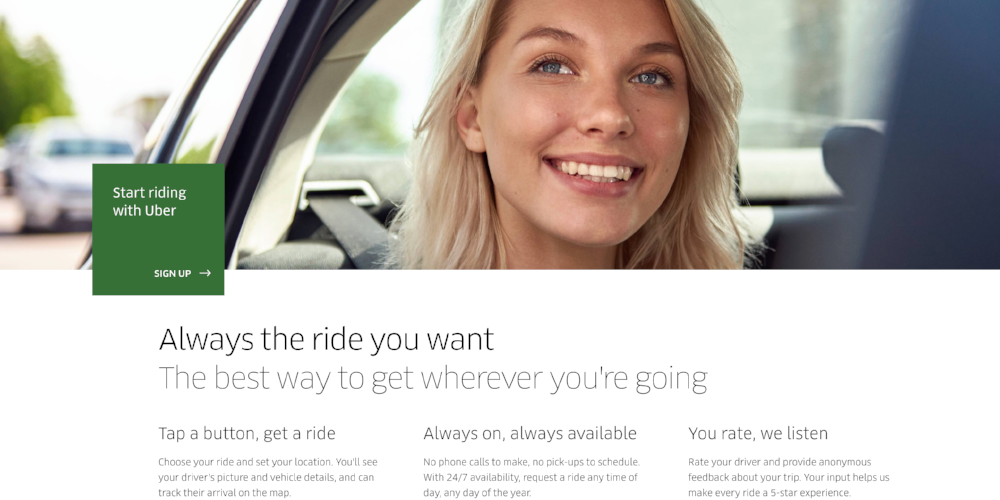The image features a close-up view of a woman sitting in a car, captured from just above her forehead down to the bottom of her neck. She has blonde hair and blue eyes, and she is smiling directly at the camera while wearing a seatbelt. In the background, there are trees and other vehicles visible through the car window. 

Overlaying the image is a green square with white text that reads "Start riding with Uber - Sign Up," accompanied by an arrow pointing to the right. Below this graphic, there is a section with a white background and large black text that says, "I'll wait the ride you want, the best way to get wherever you're going."

The text continues below, explaining Uber's features. On the left, it reads, "Tap a button, get a ride," followed by a description: "Choose your ride and set your location. You'll see your driver's picture and vehicle details and can track their arrival on the map."

Adjacent to this is another informative section that says, "Always on, always available," highlighting the convenience of the service: "No phone calls to make, no pickups to schedule. With 24/7 availability, request the ride any time of day, any day of the year."